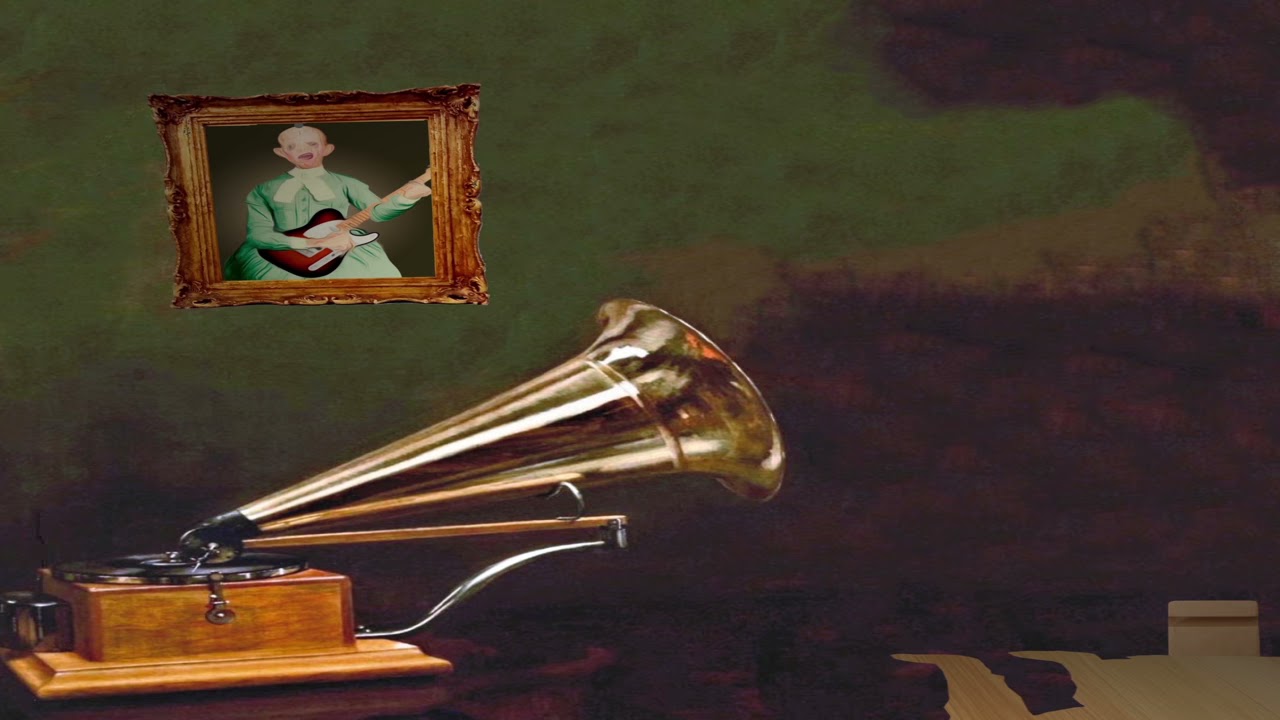The horizontally aligned rectangular image presents a collage-like scene that meshes a simulated wall with artistic elements. The background predominantly features green at the top, transitioning through a brownish rust in the middle to a dark burgundy along the bottom and the upper right corner, giving it a rich, textured appearance. In the upper left corner, there is an old-style, gold picture frame that holds an image of a person with deformed features, notably pointy ears, clad in a green outfit, awkwardly playing a guitar. Below this, in the lower left corner, stands a wooden gramophone with a black record on its turntable; its large, gold horn points towards the image's center. The lower right corner has a cream-colored shape that contrasts with the rest of the composition. The collage merges these elements to create a cohesive artistic representation, blending the realistic with the surreal.